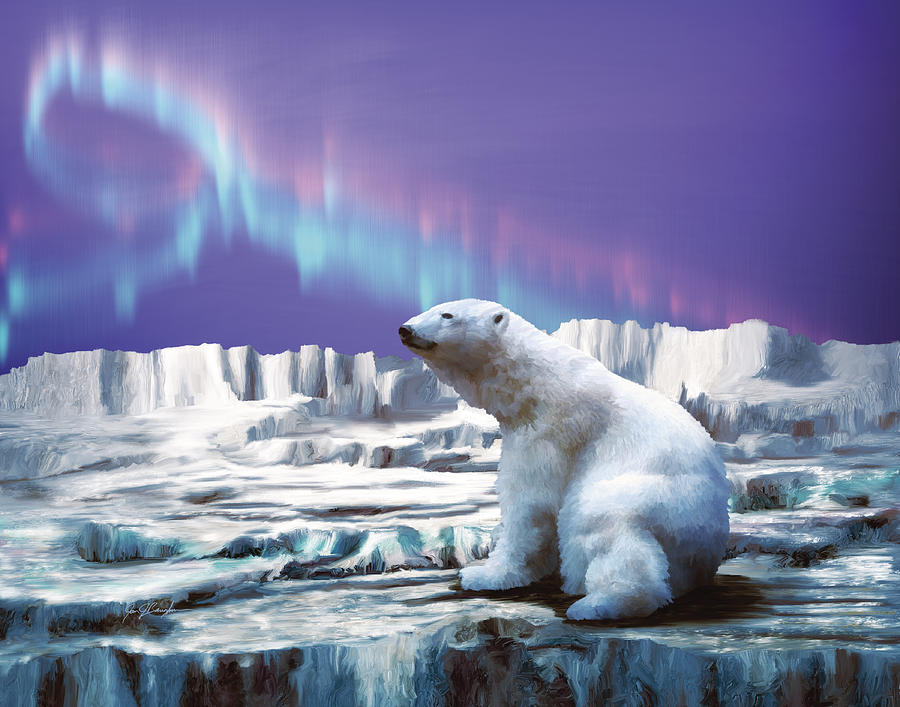In this captivating piece of artwork, a serene polar bear sits on a flat part of a melting iceberg, facing slightly left. The polar bear, with its fluffy white fur, appears peaceful as it gazes upward, seemingly admiring the sky. Behind it, the landscape is dotted with varying ice formations, from ridges to tall, greyish-white ice structures that resemble cliffs or glaciers extending into the distance. The night sky above is a stunning purplish-blue, featuring a vibrant aurora borealis that streaks diagonally from the top left to the bottom right. This aurora is composed of swirling pinks and light blues, forming a looping, circular pattern at the top left. The depiction of the ice shows signs of melting, adding to the sense of tranquility and fragility in this evocative scene.